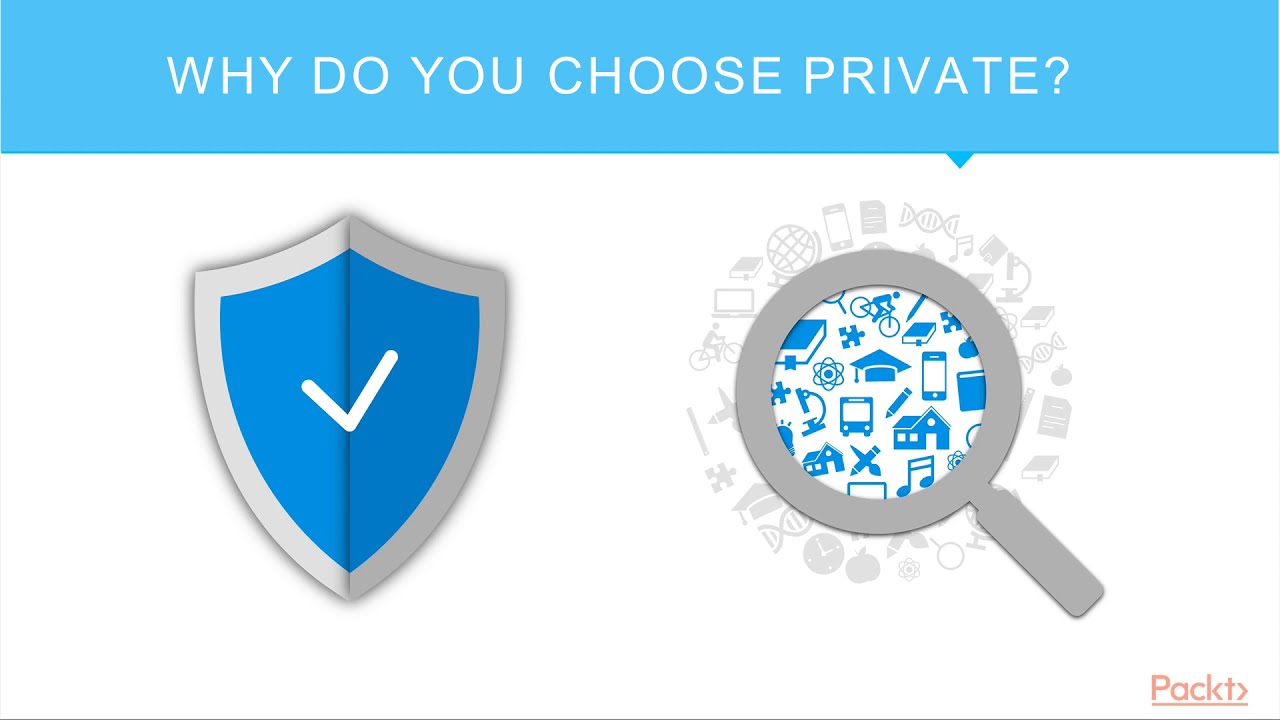The image depicts a simple graphic artwork featuring two primary icons on a white background. On the left side, there is a gray shield with a blue checkmark in the center and a silver border, symbolizing security or verification. On the right side, a gray magnifying glass hovers over various icons that represent different aspects of everyday life, such as a smartphone, a globe, a book, a laptop, a bike, a clock, and some fruit. These icons are grey outside the lens but appear blue inside it, indicating scrutiny or observation. At the bottom right of the image, the text "PACKT" is written in peach color. At the top, there's a blue rectangle with a text bubble containing the question, "Why do you choose private?", written in white text, suggesting a focus on privacy. The overall style and elements point to an advertisement likely promoting a web security or VPN service that emphasizes the importance of privacy in a world where various aspects of life can be constantly monitored.